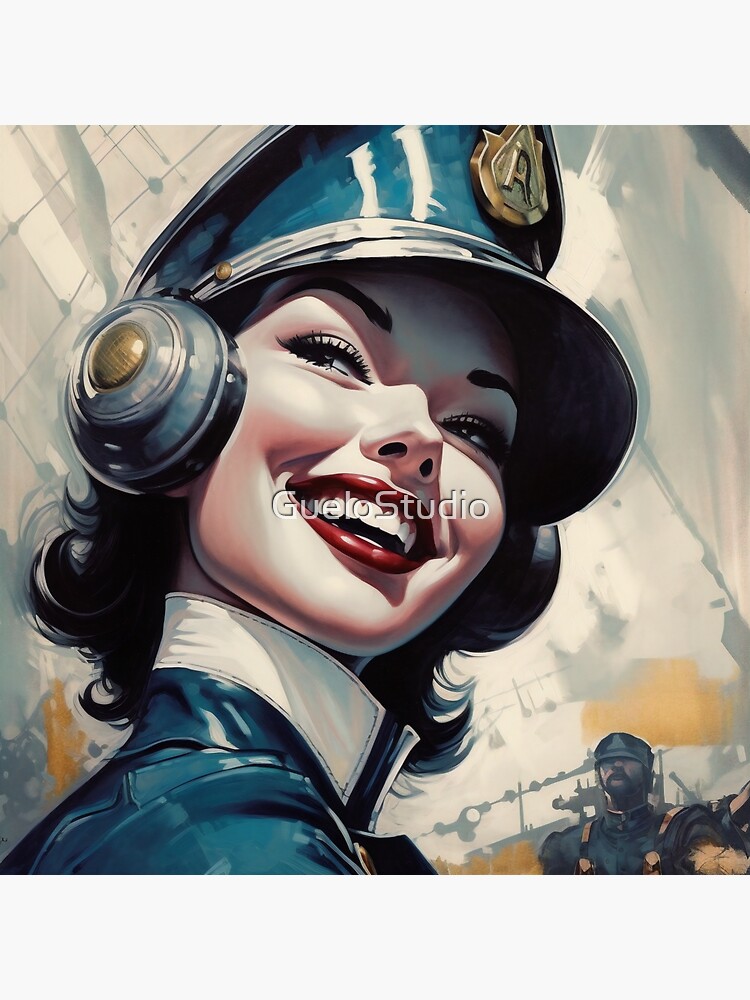This digital illustration, possibly from a game or animated show, features a detailed portrayal of a female character in a futuristic or outer space police or military uniform. She wears a blue and silver hat with a wide brim and a gold badge at the center, complemented by metallic silver, blue, and gold headphones or earmuffs over her ears. Her short, wavy black hair and dark eyebrows frame her face, which is adorned with striking red lipstick. She is smiling warmly, her eyes gazing off to the right. Her uniform, visible from the shoulders up, has a white collar and a blue top.

In the lower right corner, there is a male figure in the same uniform and hat, complete with a beard and mustache, standing in the background. The backdrop consists of splashes of yellow, gray, and white colors, adding a dynamic and somewhat abstract feel to the scene. Across the center of the image, the text "Girlo Studios" is overlaid in white, marking the creator of the illustration. 

The composition includes a noticeable light gray border on the top, lending a framed appearance to the square-shaped image. Thin gray lines in the upper left might suggest additional structural elements, though their exact nature remains ambiguous.